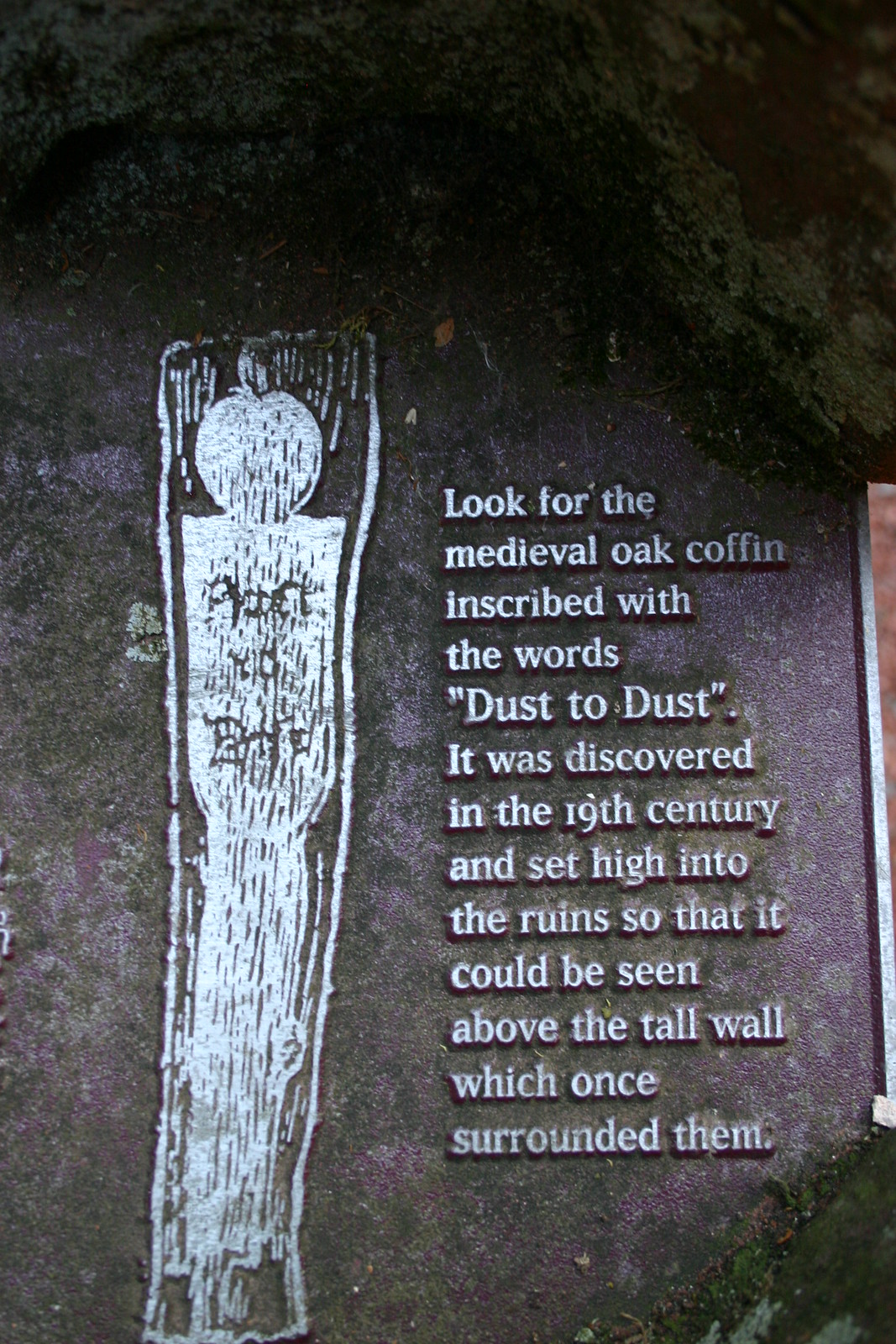The image depicts an outdoor nighttime scene featuring an old, worn rock or wooden surface that appears to bear some kind of carved or inscribed artwork. The object is set on an outdoor, grassy surface that may also contain patches of greenish moss. Central to the image is a large white vertical symbol that vaguely resembles a person—with a round, apple-shaped head tapering downwards towards a narrow waist—etched or drawn onto the rock. Accompanying this figure, on the right side of the image, is a series of white inscriptions which read: "Look for the medieval oak coffin inscribed with the words, 'Dust to Dust.' It was discovered in the 19th century and set high in the ruins so that it could be seen above the tall wall which once surrounded them." The colors in the image primarily consist of black, white, shades of green, gray, and tan.